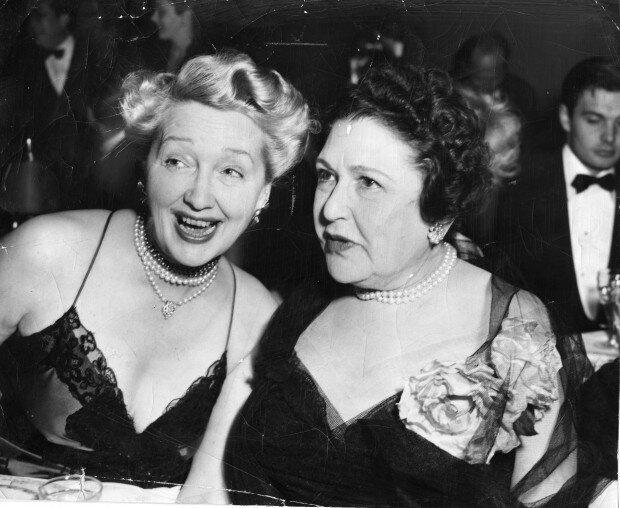This black-and-white photograph, likely taken between the 1930s and 1950s, showcases two middle-aged women, both dressed formally in black dresses and adorned with pearl necklaces. The blonde woman on the left appears highly amused, while the brunette with dark, curly hair seems to be in awe. Their hair is stylishly done up, reminiscent of the Marilyn Monroe era. Seated at a table with drinks in front of them, they are the focal points of the image. Behind them, a number of men dressed smartly in tuxedos with bow ties can be seen, slightly out of focus. The photograph, exhibiting signs of age such as scratches and creases, captures a moment of apparent fascination and elegance.